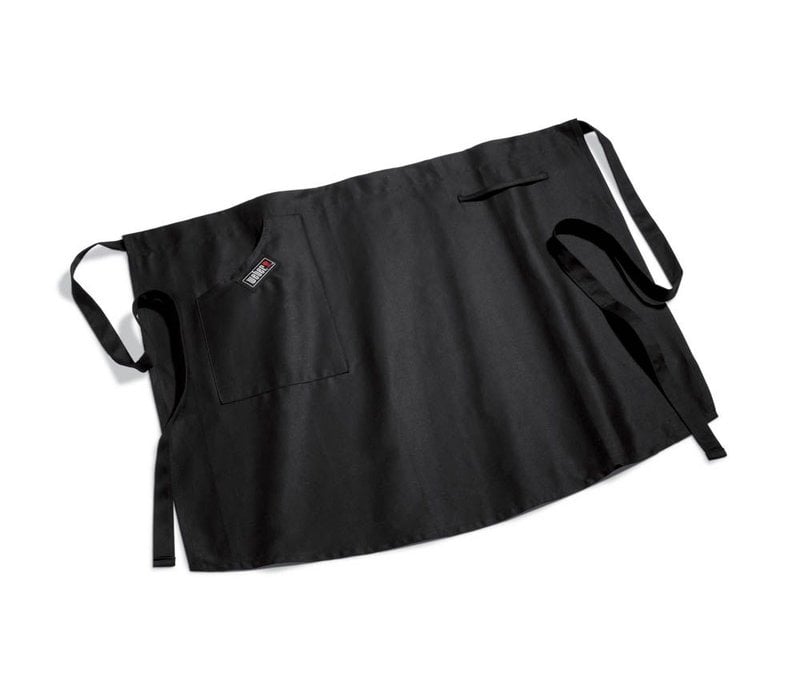The image displays a black half-apron, designed to cover the waist and lower body, laid out on a white surface. The apron, resembling a skirt in shape with a rounded bottom edge, is equipped with black ties for securing around the waist. It features a pocket on the left side adorned with a logo that includes a black box with a white border and the word "Weber" spelled out in white letters. Within the logo, there's a small red object, indicative of the Weber Grills branding. On the right side, a black string is attached at both ends, possibly used for holding utensils or other items. The apron casts a shadow on the white background, adding depth to the image.